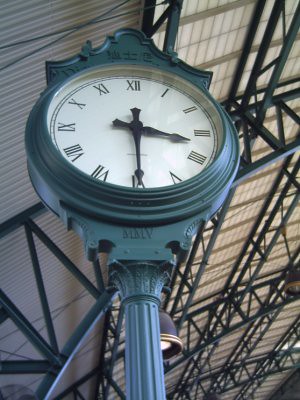In this detailed image, the viewer's perspective is from the ground looking upwards at an ornate black cast iron or steel pole. Atop this elegant post is an intricate metal frame surrounding a vintage clock reminiscent of those found in British train stations. The clock, encased in a green decorative border with alternating pointed edges resembling leaves, features a pristine white face with Roman numerals. The time indicated is 3:30, with two black hands—the minute hand pointing to six and the hour hand between three and four. A glass cover protects the clock's face, adding to its classic appearance.

The setting appears industrial with an overhead tan ceiling structured by numerous black steel girders. These girders, some arched and curved, stretch from the top-right corner to the bottom-center and from the lower-left to the right-center, mimicking the frame of an archway. Additionally, a black steel light fixture hangs from one of these girders, featuring a white bulb at its center, just behind the base of the ornate post. The ceiling, marked by its metallic slats and supported by exposed beams running both vertically and horizontally, emphasizes the rugged industrial atmosphere of the scene.